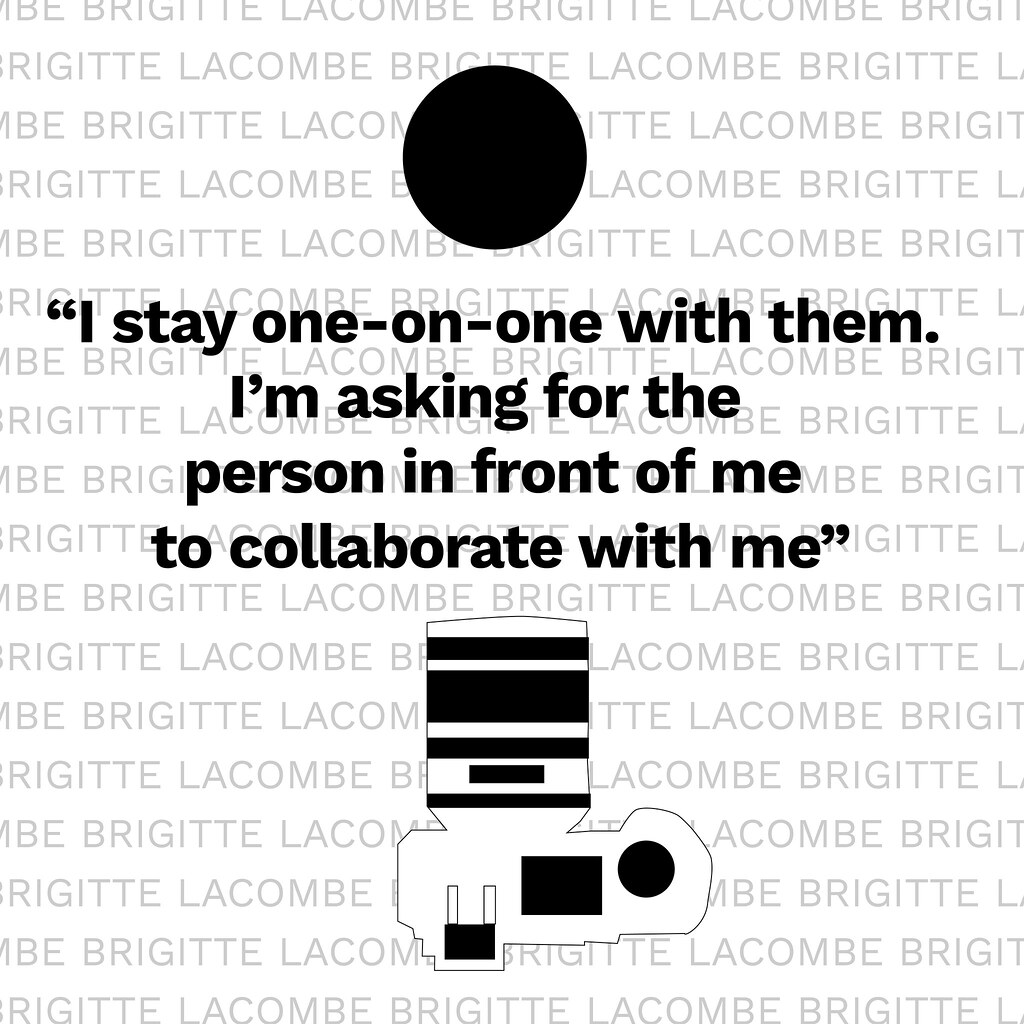The image features a light background with the words "Bridget, Look Home" and "Lacobi Bridgety" repeatedly printed in a light tan color. At the top center, there is a prominent black circle. Below this circle, a quotation reads: "I stay one-on-one with them. I'm asking for the person in front of me to collaborate with me." Further down, the image includes a complex drawing that somewhat resembles a machine or an object with black and white lines. The drawing has a horizontally elongated section with vertical black stripes, and a vertically elongated section with horizontal black stripes. In the bottom section, there are two black rectangles and a black circle. Additionally, at the bottom left, there is a socket with two protruding legs. On the right side of the image, there is another black rectangular shape.